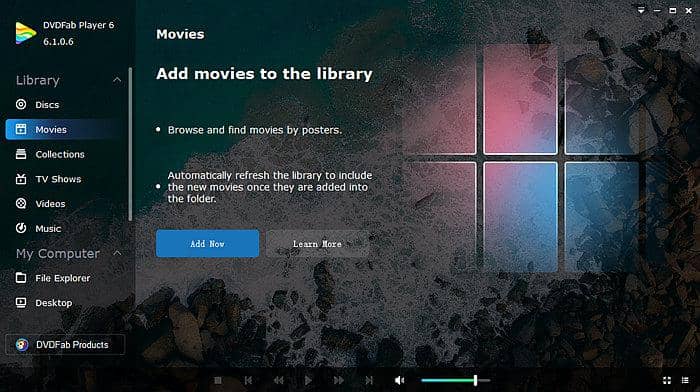This is an image of the DV-DFAB Player 6 interface. The main screen prominently offers options to "Add Movies to the Library," "Browse and Find Movies by Posters," and "Automatically Refresh the Library to Include New Movies." The interface features a prominent blue "Add Now" button and a "Learn More" link that subtly fades into the background. The backdrop for the interface is a window with visible dividers, revealing an outside view of pink-hued foliage with shades of black and brown, against a partially blue sky. The remainder of the background consists of intricate black designs on gray and black panels. To the left of the main image, a sidebar lists library categories, including Discs, Movies, Collections, TV Shows, Videos, and Music. Below this, in gray text, are options such as My Computer, File Explorer, Desktop, and DV-DFAB Products.